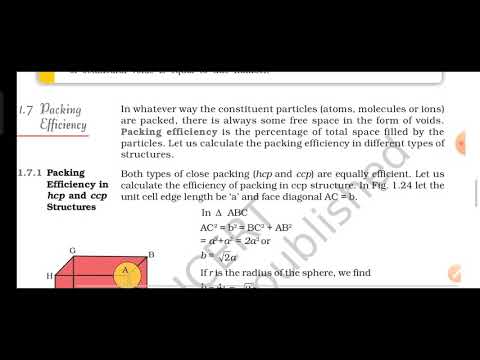The image appears to be a photograph of a textbook page against a black background, possibly with some areas redacted. At the top left of the white page is the heading "1.7 Packing Efficiency," followed by the sub-heading "1.7.1 Packing Efficiency in HCP and CCP Structures." To the right, two paragraphs explain that the packing efficiency measures the percentage of total space filled by particles, noting that there is always some free space known as voids. The first paragraph ends with an invitation to calculate packing efficiency in various structures, while the second paragraph asserts that both HCP (hexagonal close-packed) and CCP (cubic close-packed) structures are equally efficient, and introduces a calculation for CCP structures as shown in figure 1.24. This is followed by a detailed mathematical problem discussing unit cell edge lengths and sphere radii, some of which is partially cut off. 

There is a prominent red box in the bottom left corner of the page, containing an illustrative diagram labeled with letters A, B, C, and H, and a circle highlighted in orange centered at letter A. Diagonally across the image, from bottom left to top right, the gray watermark "CERT PUBLISHED" is visible. The image has a yellow text bar at the top left, although its content is obscured. A narrow black border outlines the top and right of the image, enhancing the focus on the central text and diagrams.